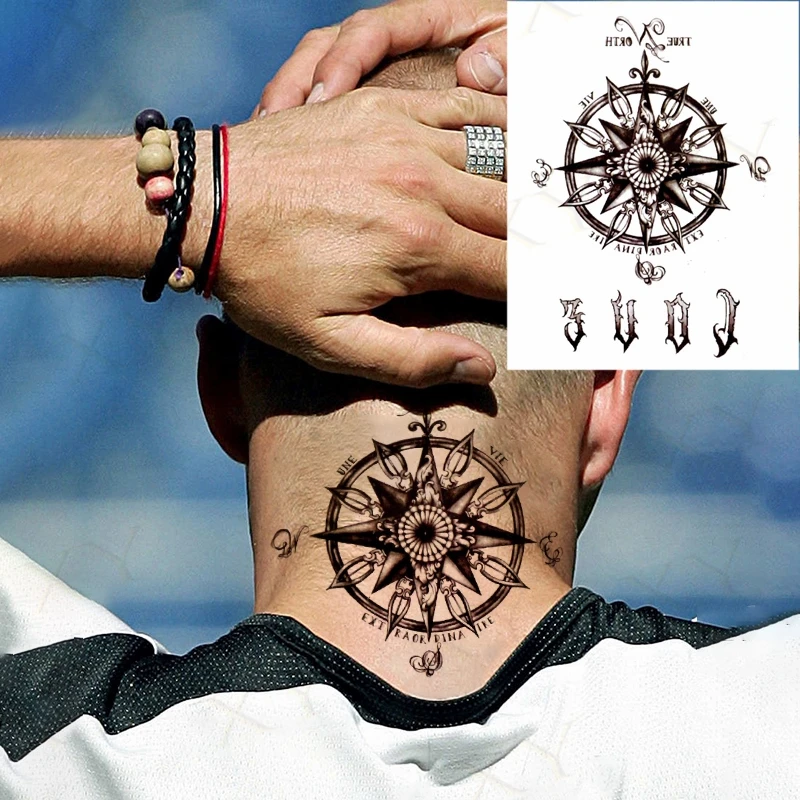In the image, we see the back of a bald man’s head and neck, adorned with an intricate, black ink tattoo resembling a Celtic compass. The man, with pale skin, faces away from the viewer, placing his left hand on the back of his head and his right hand on top of his head, showcasing a variety of bracelets on his left wrist. These bracelets include a thin, intertwined leather piece, a black and red band, and a beaded bracelet with black, green, and pink beads. On his ring finger, he wears a distinctive diamond ring with four channel-set diamonds.

The tattoo on his neck features a central star, with the cardinal directions—North, South, East, and West—marked outside the compass. The text around the compass appears to be stylized Latin, reading “UN V EXT RAUCH RINA EXT,” along with additional directional markers like North North East, South South East, North North West, and South South West, each indicated by a pointer resembling the tip of an old-fashioned pen nib.

He is dressed in a black and white shirt with black trim at the shoulders, merging into a black mesh lower down. The background of the photo is a light blue sky with white elements, enhancing the stark contrast of the tattoo and his attire. An inset image in the top right corner on a white background provides additional details of the tattoo, including more intricate text and design elements.